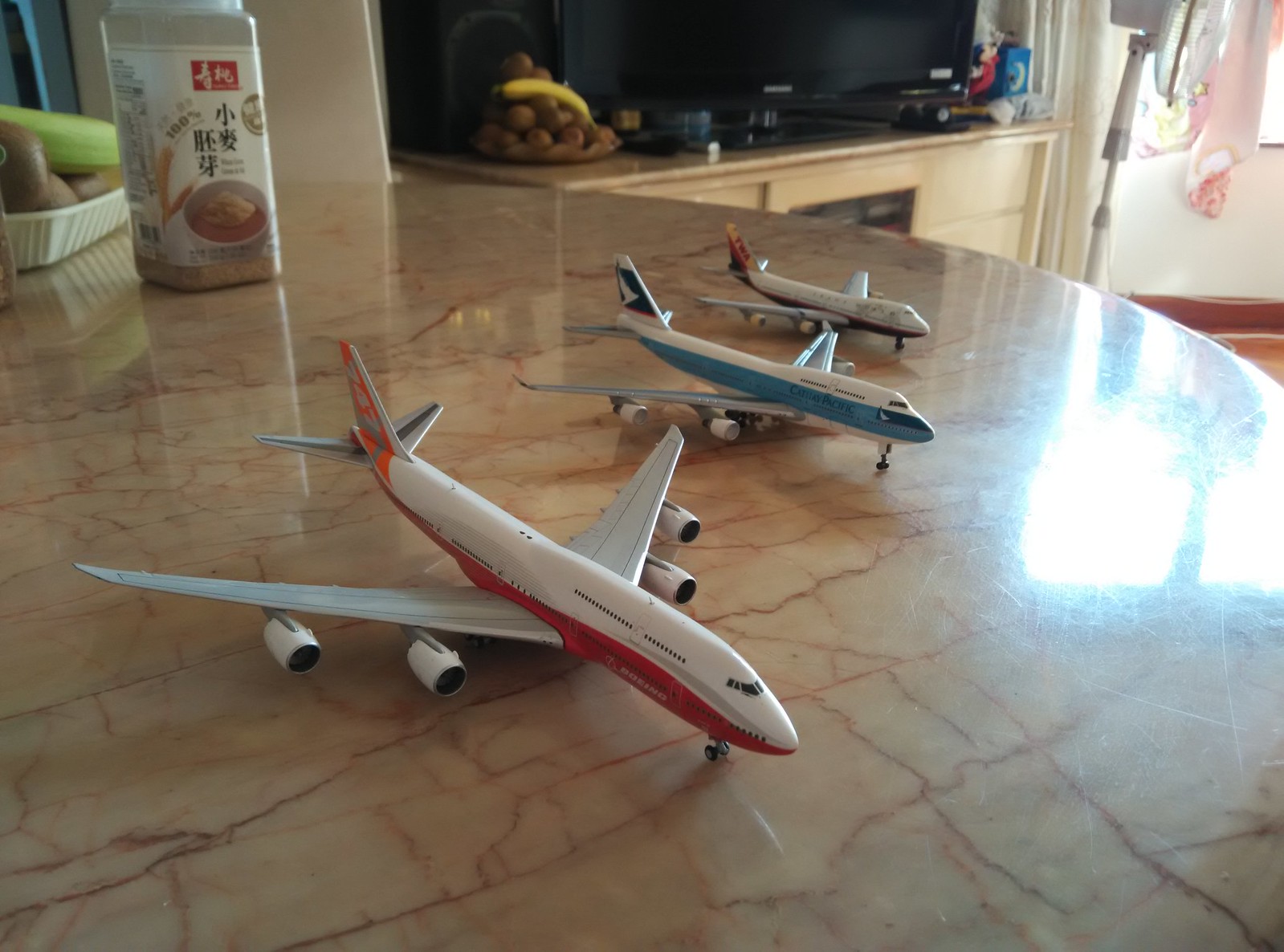In this detailed color photograph taken indoors, we see a close-up view of a round table with a beige, marbled surface featuring dark red and light brown veining, resembling granite. The focal point of the image is three model airplanes arranged from the foreground to the background. All three models are predominantly white, each distinguished by unique colorful accents: 

- The nearest airplane has a red stripe with a red tail, although some descriptions suggest an orange tail.
- The middle airplane features a blue stripe with a dark blue tail.
- The farthest airplane seems to have a dark blue or black belly with a brownish or possibly an orange tail.

The table also holds several other items. Toward the back, there’s a food container with Asian text, possibly resembling a Pepperidge Farm cookie package. To the upper left, there's a reflection of a light source on the table, indicating sunlight possibly streaming through a window with a blue curtain. Additionally, there is a shallow white ribbed dish containing a brown and a green object, potentially kiwis or a cucumber.

In the background, the setting appears to be a kitchen. We can see cream-colored kitchen cabinets, a stove with a cream enclosure, and various kitchen items, including a pile of brown fruit and a banana. There seems to be another container with some food items and utensils that are not distinctly identifiable. A piece of clothing or a cloth is draped in the upper right corner, adding to the domestic atmosphere of the kitchen space. Overall, this image combines elements of a hobbyist’s collection with a snapshot of everyday kitchen life.